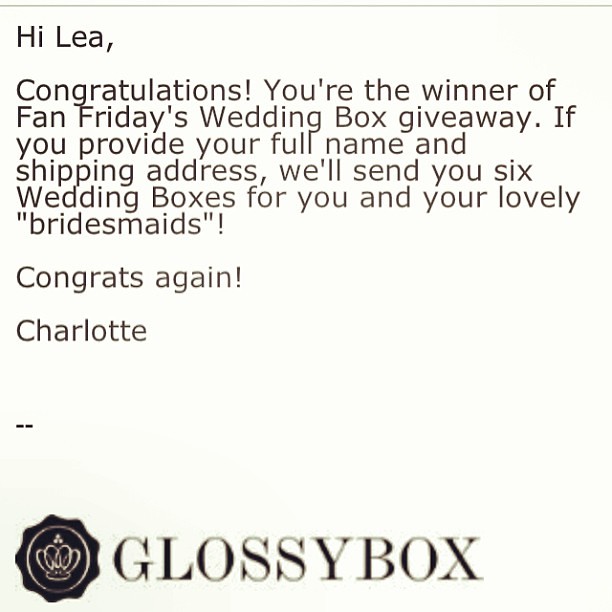The image depicts a neatly formatted letter addressed to someone named Leah. The letter opens with a friendly greeting, "Hi, Leah," and is sent by Glossy Box, which is prominently mentioned at the bottom of the letter. Glossy Box's logo, which is round with a striking black background and a white crown in the center, is also displayed in this section. 

In the main body of the letter, Leah is congratulated for winning the Fan Friday's wedding box giveaway. The letter requests Leah to provide her full name and shipping address, so that Glossy Box can send her six elegantly curated wedding boxes intended for her and her bridesmaids. The message concludes warmly with "Congrats again," signed off by someone named Charlotte.

The letter is presented on a stark white sheet of paper with clear, black fonts, maintaining a minimalist yet elegant aesthetic. The contrast between the black text and the white background, along with the highlighted black and white Glossy Box logo, makes the letter visually appealing and easy to read.